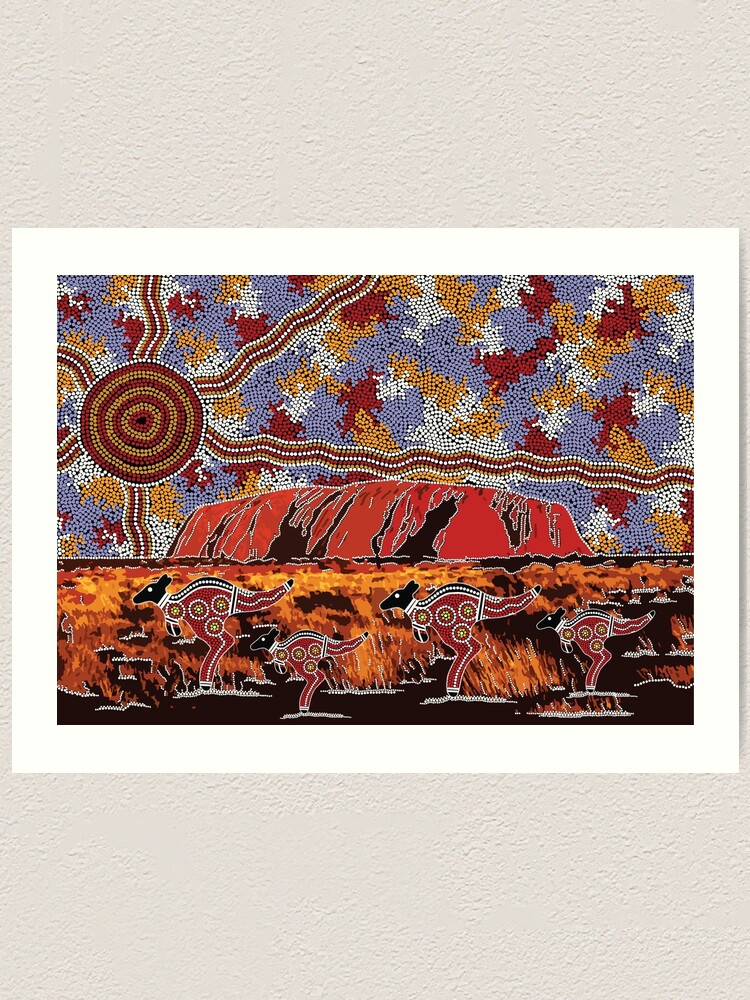This detailed piece of art, which appears to be mounted on an ivory-colored, slightly textured wall, is framed with a white mat against a white plaster background. The multicolored artwork, resembling beaded or dotted art, vividly depicts the Australian Outback. In the foreground, four stylized kangaroos—two large and two smaller—are in mid-gallop, characterized by their black heads and red bodies adorned with intricate geometric shapes. The shapes include four white-outlined circles with red centers, yellow rings, and white dots in each circle. The kangaroos seem to be leaping through a field that’s either on fire or illuminated with an intense orange hue, potentially representing the arid desert landscape. Above the kangaroos, a red rock formation, likely Uluru, stands prominently, reflecting the stylized sun's radiance. The ornate sun, crafted with spiraled bead designs in blues, reds, yellows, and whites, sends out tendrils that resemble a series of pins radiating light across the sky. This piece effectively uses beaded patterns to generate a contrast-heavy, textured landscape, capturing the essence of Australia’s unique terrain and vibrant wildlife.